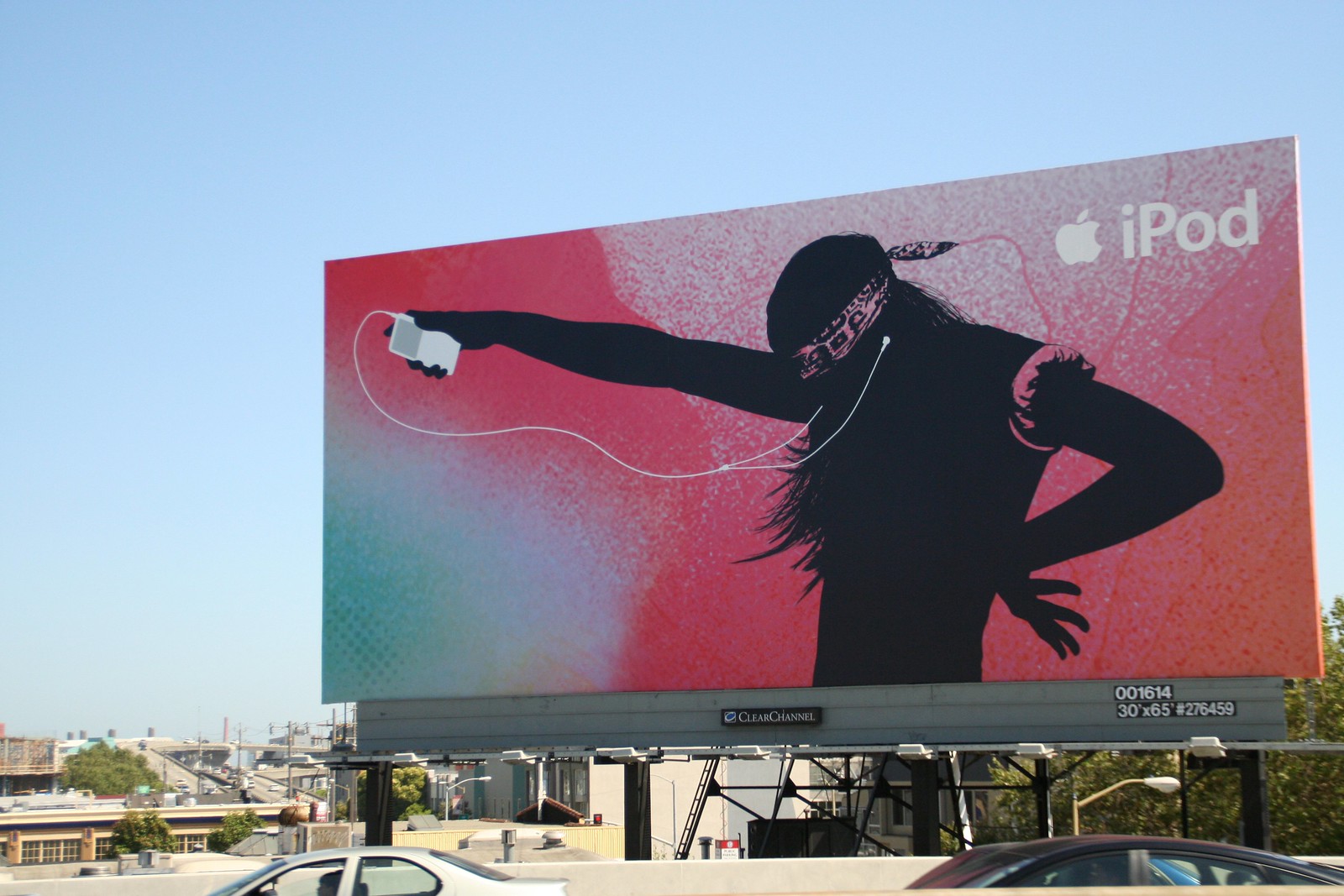The photograph captures an outdoor scene under a clear, gradually lightening blue sky. Central to the image is a large billboard set against a background that includes a highway system with a few visible cars, including a white sedan on the left and a darker, possibly black sedan on the right. The billboard dominates the middle portion of the image, situated above a small black rectangle bearing the name "Clear Channel."

The billboard itself features a vibrant design with a predominantly purple background that fades to a lighter color at the top, contrasted by hints of blue and green at the bottom left. It prominently displays the word "iPod" alongside the Apple logo at the top. The main visual element on the billboard is a black silhouette of a person with long hair, adorned with a pink bandana tied around their head and a t-shirt with puffy sleeves that are rolled up to the shoulder. The silhouette is depicted with headphones in their ears, connected by a wire to an iPod held in their outstretched right hand, while their left arm is bent with the wrist resting on their waist. The detailed features of the billboard and the surrounding elements create a vivid and dynamic outdoor advertisement scene.